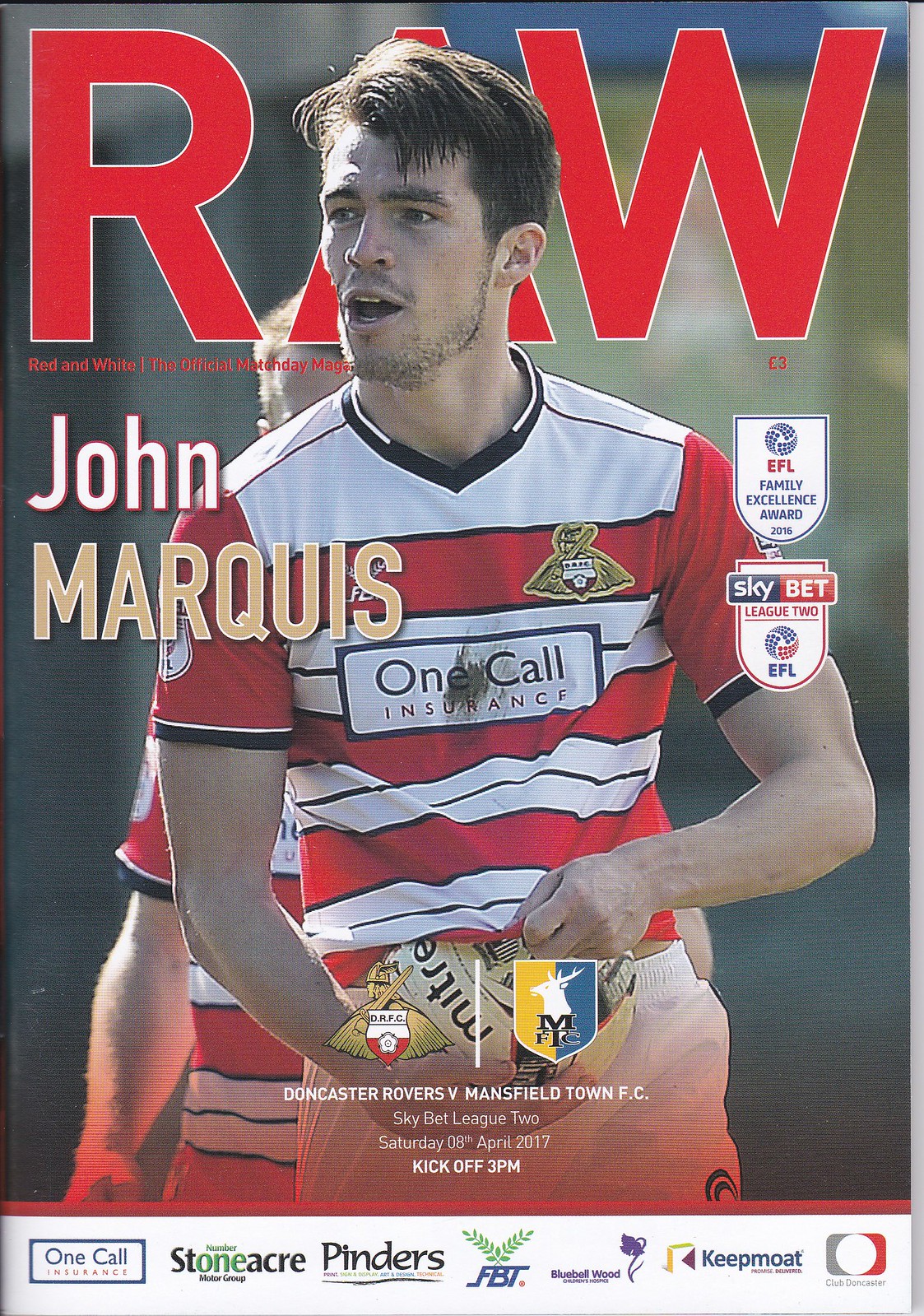The front cover of this soccer magazine prominently features a young man named John Marquis, dressed in a red and white striped jersey with a white collar. The jersey displays the 'One Call Insurance' logo in a rectangular box on the chest, with the football club's emblem positioned above it. Above Marquis’s head, the title of the magazine, "RAW," is written in large red letters, though the 'A' is partially obscured by his head.

Marquis stands with his hands in front of him, looking to his right. Over his left shoulder, there are symbols for Sky BET and the EFL, along with a Family Excellence Award medallion. Below his image, the text announces a match: "Doncaster Rovers vs. Mansfield Town FC," scheduled for Saturday, 08 April 2017, with a kickoff at 3 pm. 

At the bottom of the cover, several sponsors are listed sequentially: One Call, Stone Acres (misread as DonateCare in one caption), Pinders, FBT, and Keep Moat. The lower-right corner features a distinctive square with a red border on the right and a gray border on the left.